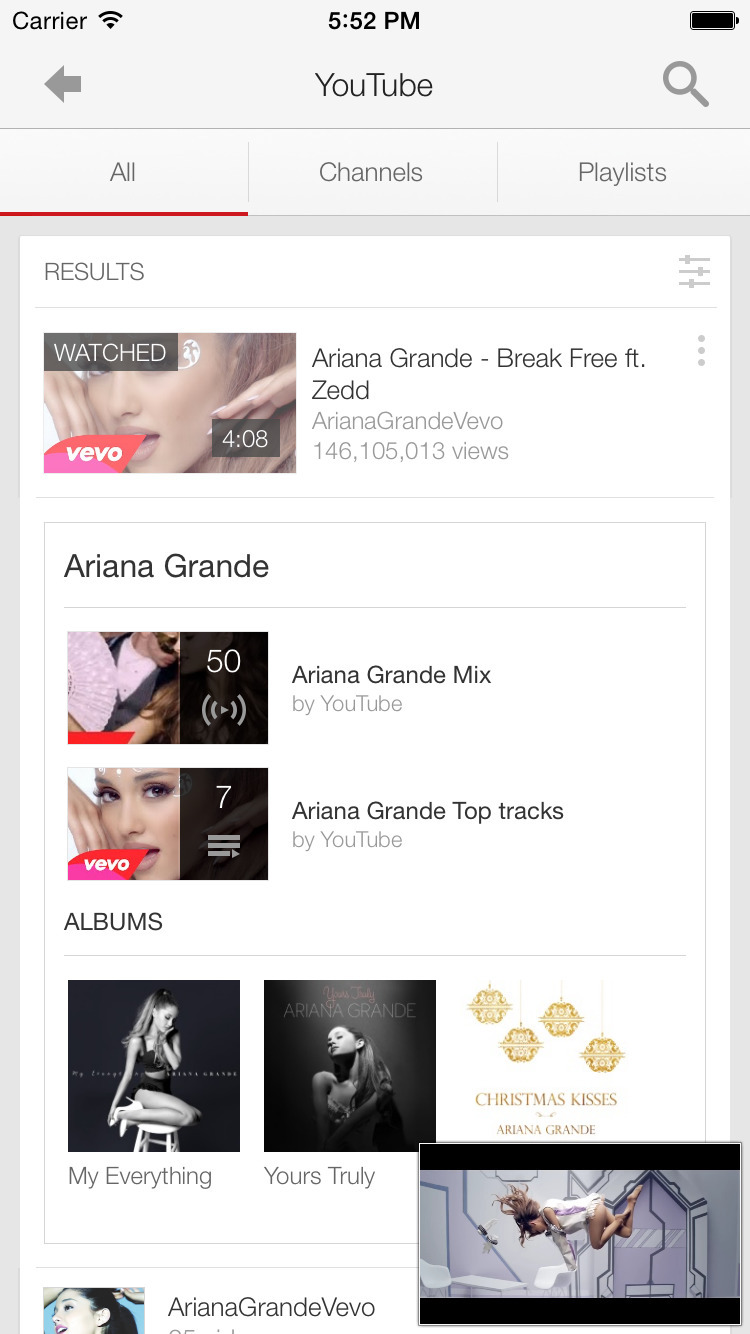**Detailed Caption:**

This screenshot, captured against a white background, details a YouTube search interface at 5:52 PM. On the top-left corner, it shows a left arrow and a magnifying glass icon. The search results are categorized under "All," "Channels," "Playlists," and "Albums," with the "All" category underlined in red. 

Prominent among the results is the music video for "Break Free" by Ariana Grande, featuring Zedd, marked as "watched." The video thumbnail is displayed, showing a duration of 4 minutes and 8 seconds. Below the thumbnail, it lists "ArianaGrandeVevo" as the channel name, with an impressive view count of 146,105,013 views.

Further down, the search results include a curated "Ariana Grande Mix," represented by an image with "50" overlaid on it. Following this, another thumbnail with "7" overlaid on it represents "Ariana Grande Top Tracks." Additionally, two album thumbnails are displayed: the first for "My Everything" and the second for "Yours Truly," each positioned under their respective album titles.